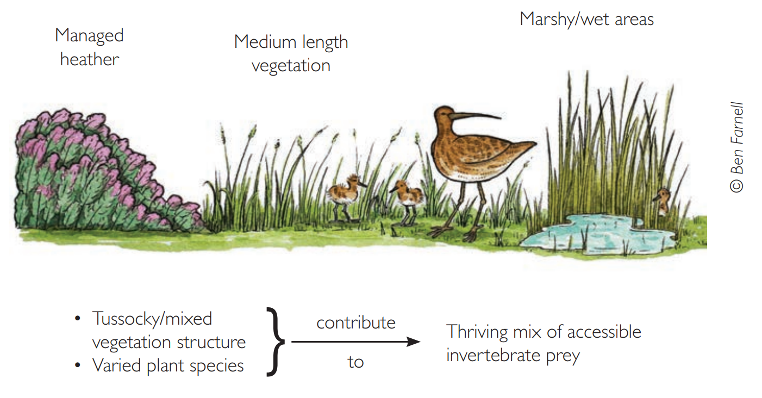This detailed illustration, likely set in the United Kingdom, features a wet, marshy area depicted with botanical precision. Central to the image is a long-billed shorebird, characterized by a grayish-brown body with brown spots on top and a white, streaked underside, complemented by long legs ideal for wading. Accompanying this bird are three chicks: two are adjacent to the parent in the center, and a third is partially hidden behind reeds on the right. The chicks resemble the adult but have noticeably smaller bills.

The background showcases a variety of vegetative elements including straight, thin-leaved reeds with flowering stems, and broad-veined leaves that culminate in purple, triangular-shaped flowers on the left. The water is rendered in light blue with white highlights, suggesting movement and depth. Text labels like "managed heather," "medium-length vegetation," and "marshy/wet areas" provide context for these plant zones.

At the bottom, the terms "tussocky/mixed vegetation structure" and "varied plant species" are noted, with an arrow indicating that these contribute to a "thriving mix of accessible invertebrate prey," essential for the ecosystem represented. The illustration is credited to "Ben Farnell," with his name vertically positioned alongside the drawing.